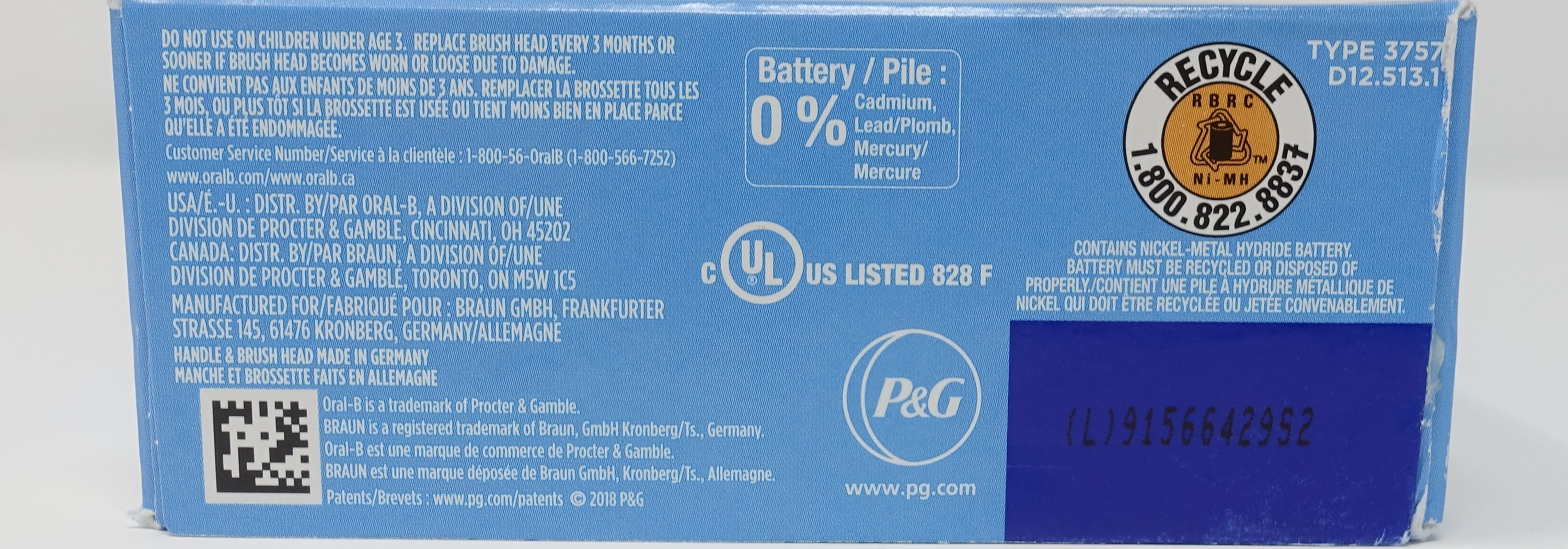This very narrow horizontal image offers a close-up of the back packaging of an electric toothbrush box. The box is predominantly a medium pale robin blue color, adorned with white text. At the bottom right corner, a large blue rectangular area features a code stamped in black ink. Most of the lettering on the back of the box is in white, providing clear and stark contrast against the blue background.

At the very top center of the box, the text reads "Battery / Pile" in reference to the power source. Directly below, it states "0% Cadmium, Lead" and "Mercury" in three different languages, emphasizing the product’s safety compliance. The package bears the UL certification mark, indicating it meets specific safety standards and is manufactured by Proctor & Gamble. In the top right corner, there is a recycling symbol, encouraging proper disposal.

On the lower right side of the box, just above the large blue area, is a prominent QR code. Below this, a warning advises, "Please do not use on children under age 8." Further instructions clarify, "Replace brush head every three months or sooner if brush head becomes worn or loose due to damage."